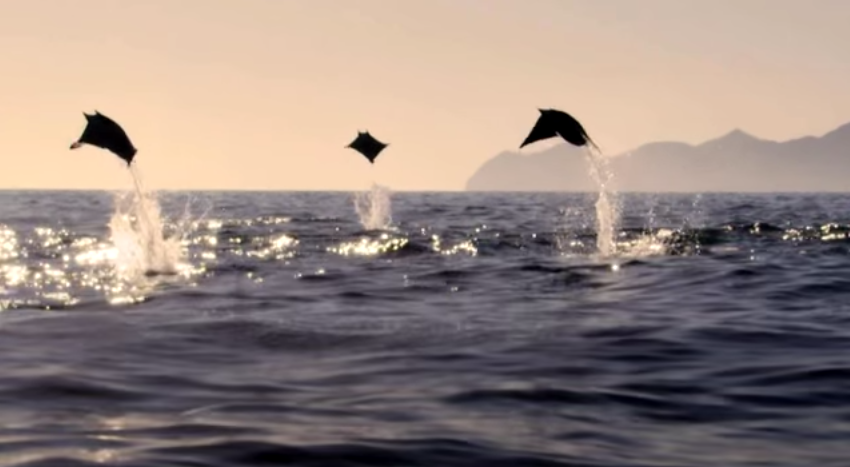In this intriguing image, we observe a vast expanse of dark blue ocean stretching across the lower half of the scene, with gentle waves creating a rhythmic pattern. Three mysterious creatures are captured mid-leap, each emerging dynamically from the water, creating noticeable splashes beneath them. The creatures are positioned from left to right. The left and right creatures resemble the shape of a horse's head with possible wing-like extensions, while the central figure takes on more of a diamond or kite shape, accentuated by its distance.

The background reveals a serene but somewhat eerie sky, painted in hues of gray and pink, adding to the enigmatic atmosphere of the scene. On the right side of the image, a faint mountain range is visible, contributing to the backdrop without detracting from the oceanic focus. Sunlight glimmers on the ocean’s surface, particularly around the splashing forms of the creatures, enhancing the visual drama of their leap. Overall, the scene combines elements of mystery and natural beauty, evoking curiosity and wonder about the origins and nature of these strange flying beings.